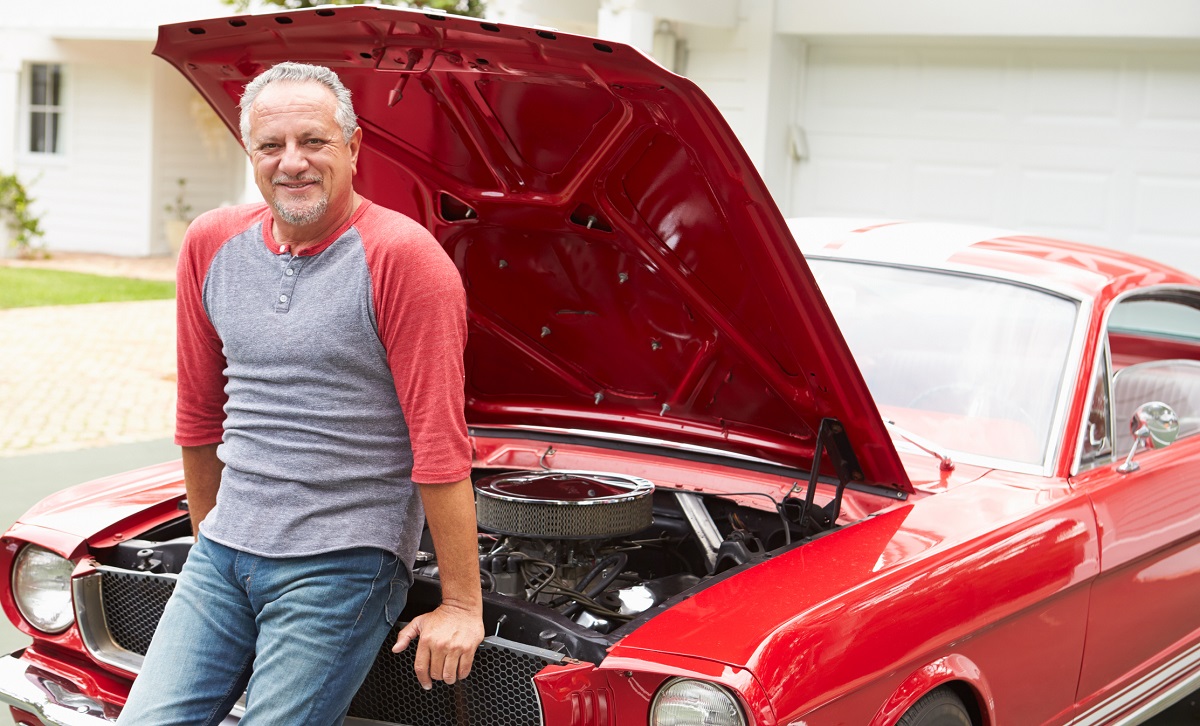This is a detailed color photograph of an older man, possibly in his 50s or 60s, leaning on the open hood of a meticulously cared-for, shiny red car, likely a 1960s or 1970s muscle car such as a Mustang or a Thunderbird. The car, gleaming from a recent buff and wax, has its left window halfway rolled down and features primarily red leather seats with white accents. The hood is open, revealing the engine and mechanical details inside. The man, with his gray hair combed back and a gray goatee, is smiling at the camera. He is wearing a gray baseball tee with red three-quarter sleeves and blue denim jeans. The background showcases a white house with an attached white garage, a muted grassy front yard, and parts of a paved driveway and walkway.